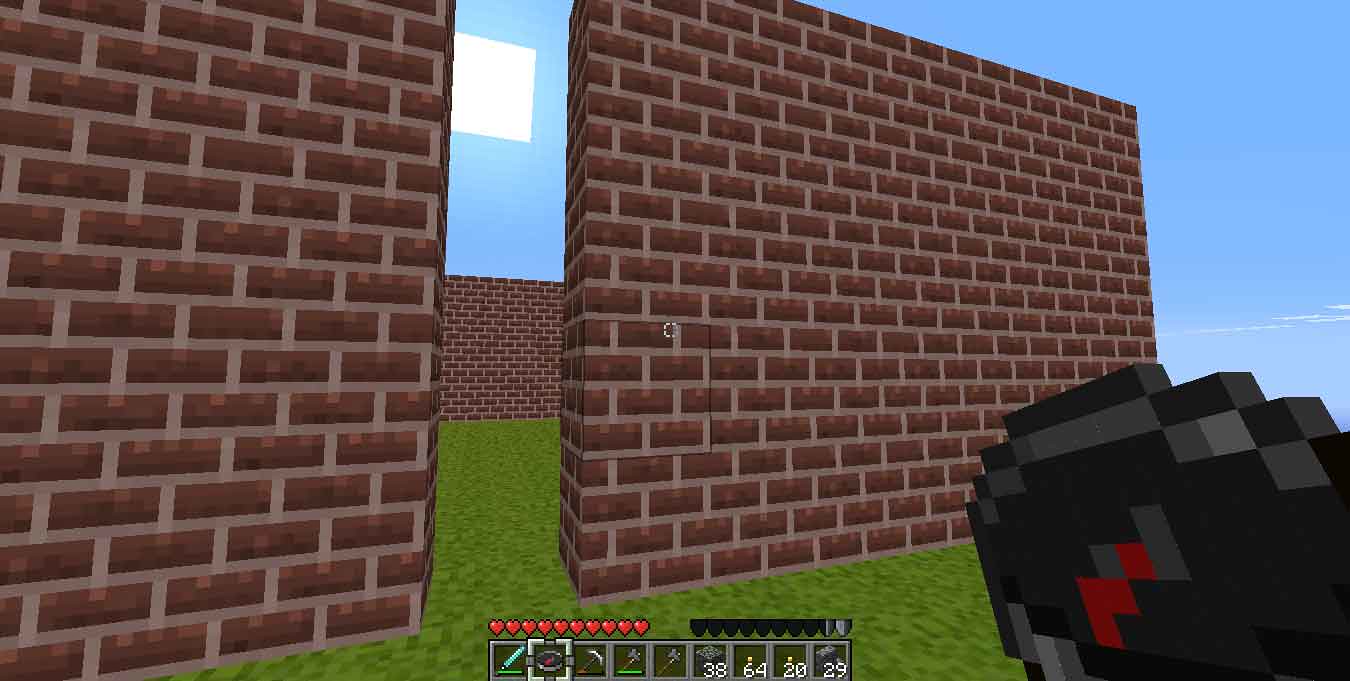The image exudes a strong resemblance to Minecraft with its distinct pixelated aesthetic. Dominating the middle center are status icons, prominently featuring pixelated hearts, some of which are illuminated in vibrant red with subtle white highlights on the upper part of the hearts. The pixel size varies, with some pixels appearing larger and others smaller, adding to the retro visual charm.

The ground beneath appears to be lush green grass, suggesting an outdoor scene. Prominent in the foreground are red brick walls, meticulously detailed with gray mortar filling the gaps between the horizontally aligned rectangular bricks. A noticeable gap is present in the wall, possibly serving as a narrow passage that may or may not be navigable. Beyond this opening, another red brick wall is discernible, indicating layered depth in the structure.

The sky transitions from a light blue near the horizon to a slightly darker blue higher up, peppered with faint clouds. A striking white square, possibly representing the sun, stands out against the sky, casting a subtle reflection that enhances the atmospheric feel. In the lower right-hand corner, an object is gripped in what appears to be the player's hand—mostly black with patches of red and gray—implying that it might be a tool or weapon within this pixelated world.